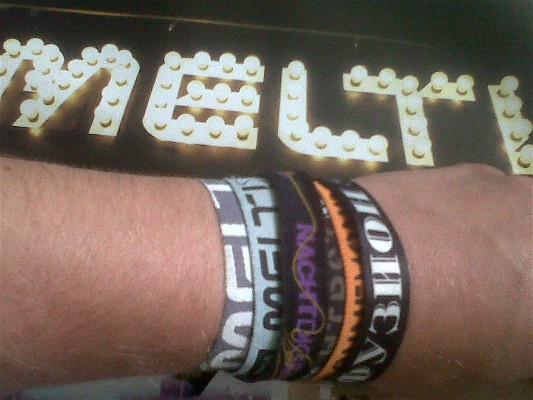This color photograph features a close-up of an individual’s forearm and wrist, adorned with numerous wristbands of different colors and materials, including rubber and paper. The wristbands, six in total, showcase a variety of languages and inscriptions, including one black band with white Cyrillic letters. Visible wristband colors include white, gray, black, purple, and orange, although some inscriptions are indistinct due to the bands being closely stacked. In the background, a vintage-style marquee with chaser lights and incandescent bulbs against a black backdrop stands prominently. The illuminated marquee displays partially visible letters "E-L-T," potentially spelling out "MELT" or a related word, with additional letters cut off on the right and left sides. The image captures the juxtaposition of the vibrant, diverse wristbands on the wrist against the glowing, nostalgic marquee lights, suggesting the setting is potentially a performance or event space.